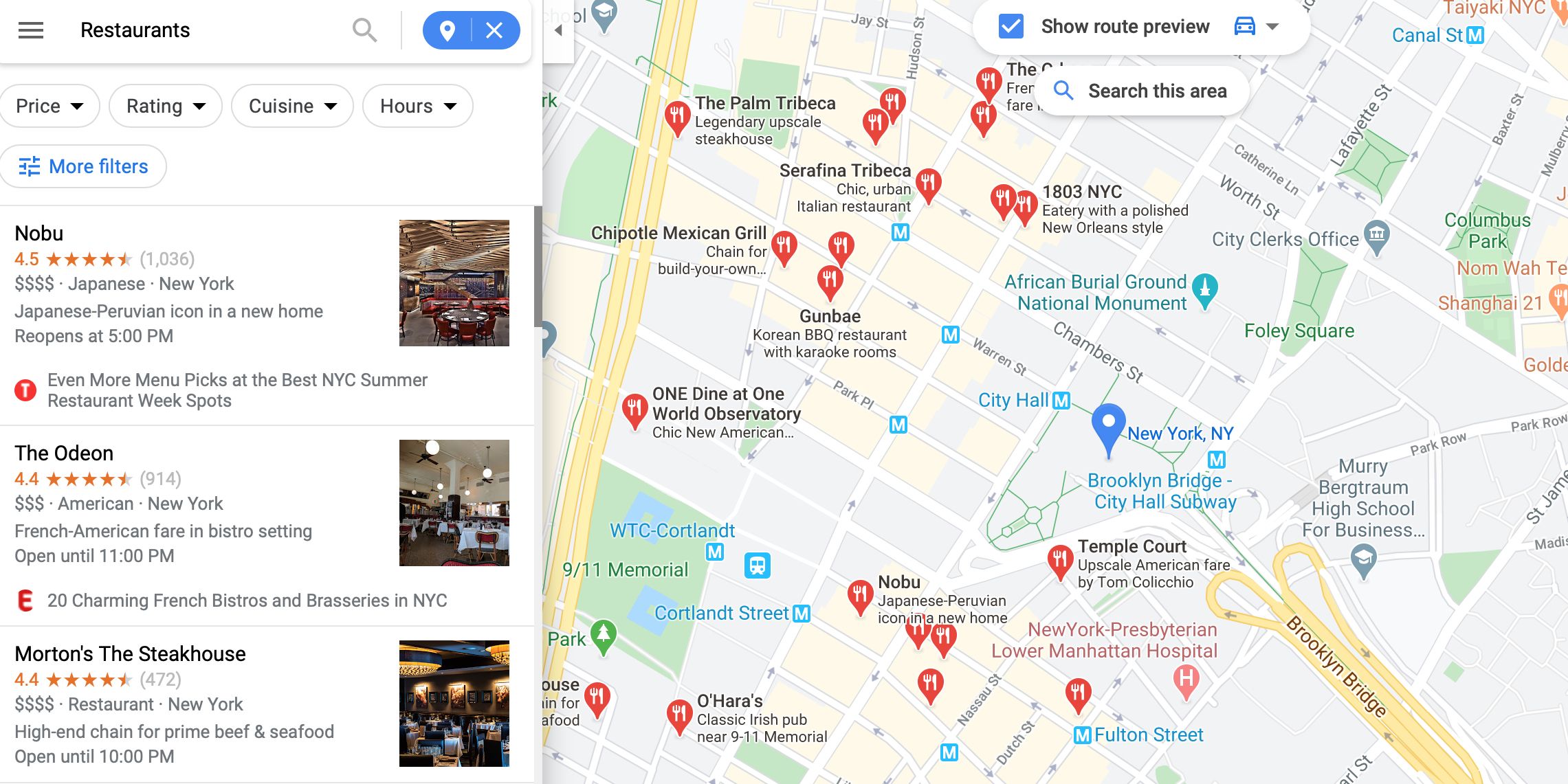A Google Maps search for "restaurants" is displayed, featuring a user-friendly interface for exploring dining options in New York City. On the left, a search bar at the top reads "restaurants," followed by filter options such as price rating, cuisine type, hours, and more. Below these filters, several restaurant listings are shown, each accompanied by a small image of the restaurant's interior.

1. **Nobu**:
   - **Image**: Interior of Nobu restaurant
   - **Description**: "Japanese-Peruvian icon in a new home"
2. **The Odeon**:
   - **Image**: Bistro-style interior
   - **Description**: "French-American fare in a bistro setting"
3. **Morton's Steakhouse**:
   - **Image**: Elegant dining interior
   - **Description**: "High-end chain for prime beef and seafood"

To the right of these listings, a detailed map of New York City is presented, highlighting notable landmarks such as the Brooklyn Bridge and various streets. The map is peppered with pins indicating the locations of various restaurants, each marked with a small fork and knife icon. The user's current location is also marked, showing their proximity to the listed dining options.